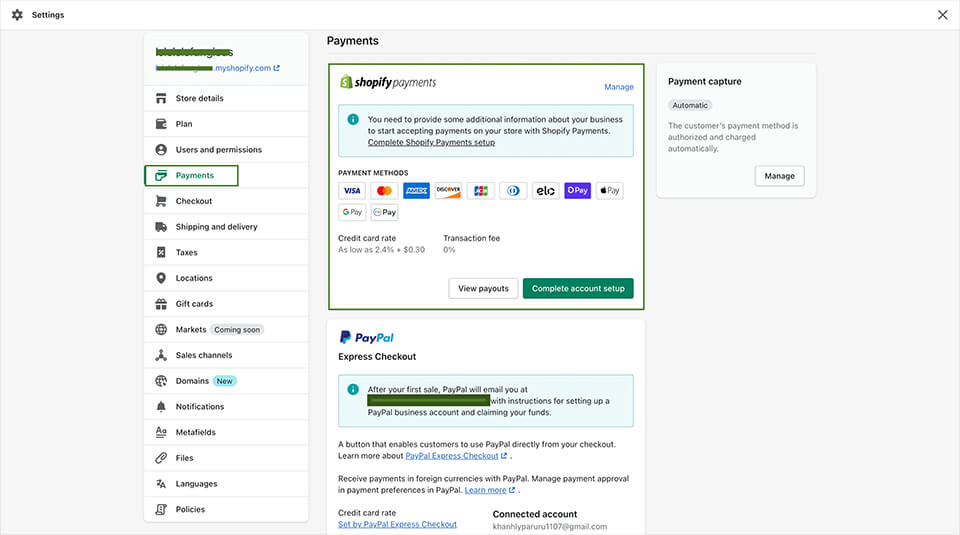The image depicts a white-backed webpage interface with various vibrant colors including blue, green, red, and orange. At the top of the page, a gear icon represents settings, while an 'X' is located in the upper right-hand corner to close the page. On the left-hand side, a vertical menu lists different sections: "Store Details," "Plan," "Users," and "Permissions," each accompanied by corresponding icons. 

There is a circular user icon next to these sections, followed by a highlighted green and blue section labeled "Payments" displaying a credit card image. Below: "Checkout" with a cart icon, "Shipping and Delivery" marked by a truck icon, and "Taxes" illustrated with a document and an X mark. Moving further down, "Locations" is signified by a pin icon, "Gift Cards" by a gift box, and "Markets," accompanied by a globe, indicating features coming soon. "Safe Channels," "Domains" (highlighted in blue), "Notifications" (marked with a bell icon), "Files," "Languages," and "Policies" follow in the menu.

In the center of the page, a green shopping bag with an "S" represents Shopify Payment Options, flanked by logos of Visa, MasterCard, American Express, and Discover. Options for alternative payment methods like PayPal, Apple Pay, and Google Pay are also available. At the bottom, a prominent green button labeled "Complete Account Setup" facilitates the final checkout process.